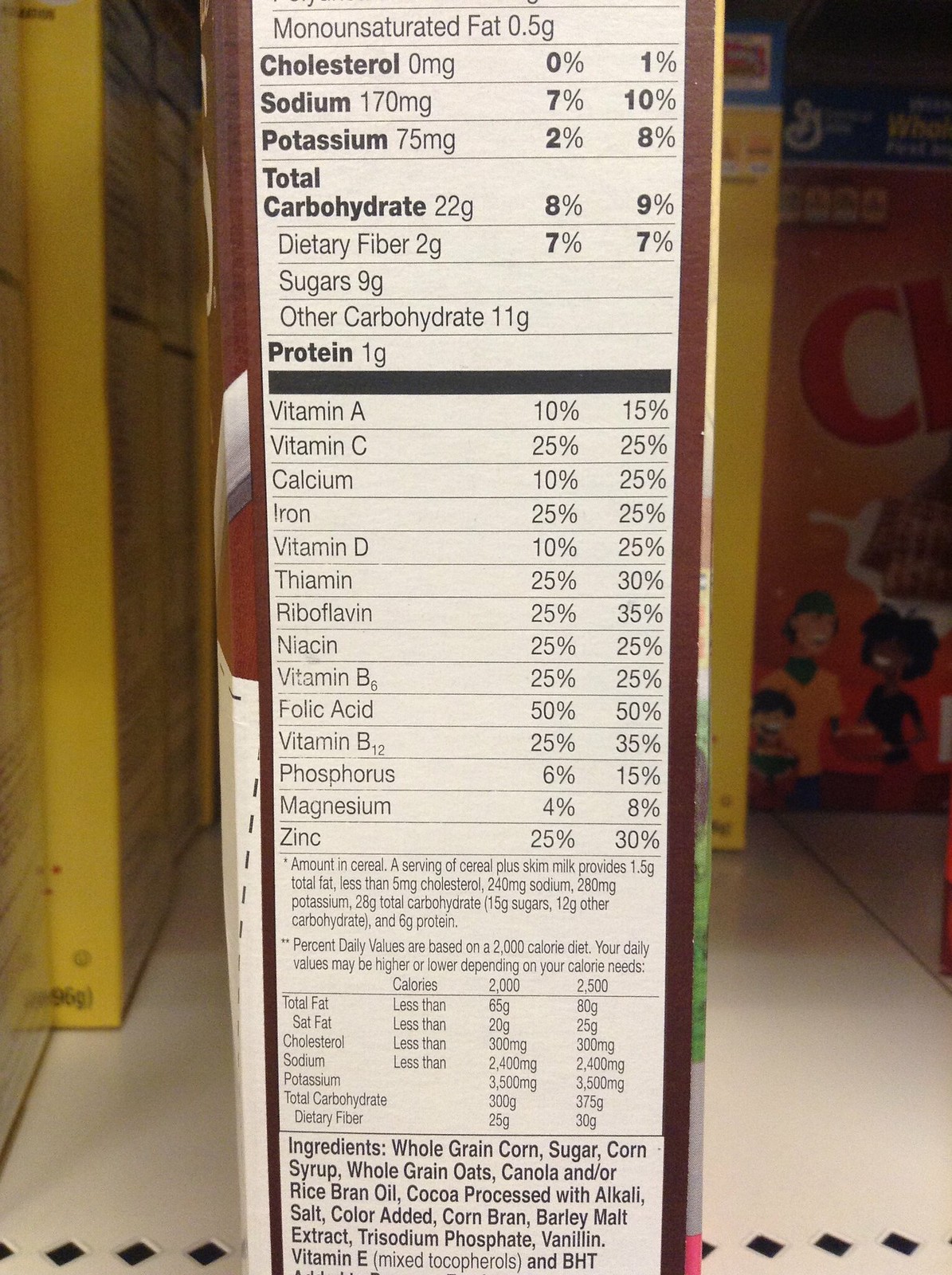Caption: 

A detailed side view of a cereal box positioned on a white retail shelf, showcasing its nutritional information clearly printed on the cardboard surface. The box features a brown border along its sides. Surrounding the central box are other cereal boxes, partially visible, primarily displaying checks and yellow colors. The shelf itself is white with a distinctive diamond-hole pattern running in a row along the front edge. The nutritional details begin with monounsaturated fat at 0.5 grams and proceed to enumerate cholesterol, sodium, potassium, total carbohydrates, fiber, and sugars. Following these are extensive lists of vitamins and minerals, along with columns indicating the recommended daily allowances. The bottom section of the box encapsulates the ingredients list.